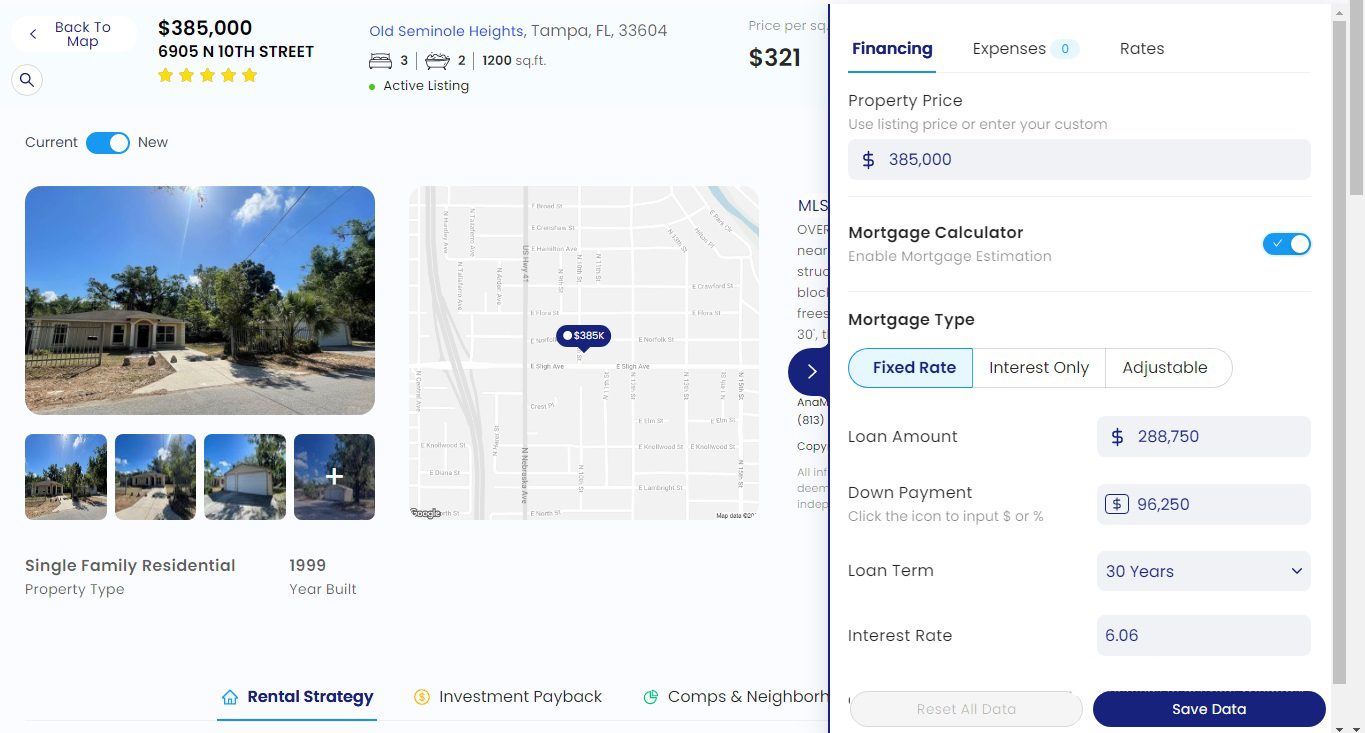This is a horizontal rectangular image displaying a detailed overview of a property listing and other related information. The left side of the image is mainly dominated by an off-white background. At the top left-hand corner, there is a small white area with the text "Back to map" in black font. Adjacent to it, the bold black text displays "$385,000."

Below, the address "6905 N 10TH STREET" is prominently featured in all caps, accompanied by five yellow stars indicating a rating. Further down, you see the words "Current" on the left side and "New" on the right side, with a button in between that is shifted to the right, displaying a turquoise color on the left side.

The center of the image includes a larger horizontal rectangular picture showing a blue sky, green trees, and a modest house. Below it, four smaller vertical images are displayed, though they are too tiny to distinguish any details.

On the left side under these images, the text "SINGLE FAMILY RESIDENTIAL" appears in all caps and black font, followed by "1999" indicating the build year. Beneath these, "property type" is noted next to "year built." Towards the bottom left, "Rental Strategy" is highlighted in blue font with a turquoise underline and a small turquoise house icon next to it. Next to this, "Investment Payback" is written, followed by the words "Comps" and "Neighborhood" with small icons preceding them.

Adjacent to the images, a map is displayed on the right side of the page.

At the upper right of the page, the word "Financing" is in dark blue font and underlined with turquoise. Below this, the word "Expenses" appears next to a turquoise oval containing a zero. Underneath, the section lists "Rates" followed by "Property Price." It allows you to "Use listing price or enter your custom" value, with a pre-filled light gray horizontal space showing "385."

Beneath this, "Mortgage Calculator" in bold black font appears, with an option to "Enable mortgage estimation" that is toggled on, signified by a turquoise button with a white check mark. The "Mortgage Type" section offers three options in a horizontal line separated by gray lines: "Fixed Rate" highlighted in a light blue area with dark blue writing, "Interest Only," and "Adjustable" in light black text.

In the "Loan Amount" section, a space shows "$288,750." The "Down Payment" area lists "$96,250," followed by "Loan Term," set at "30 years" with a small down arrow on its right. The "Interest Rate" is marked as "6.06." Finally, at the bottom, a "Save the Data" button is displayed in dark blue with white writing.